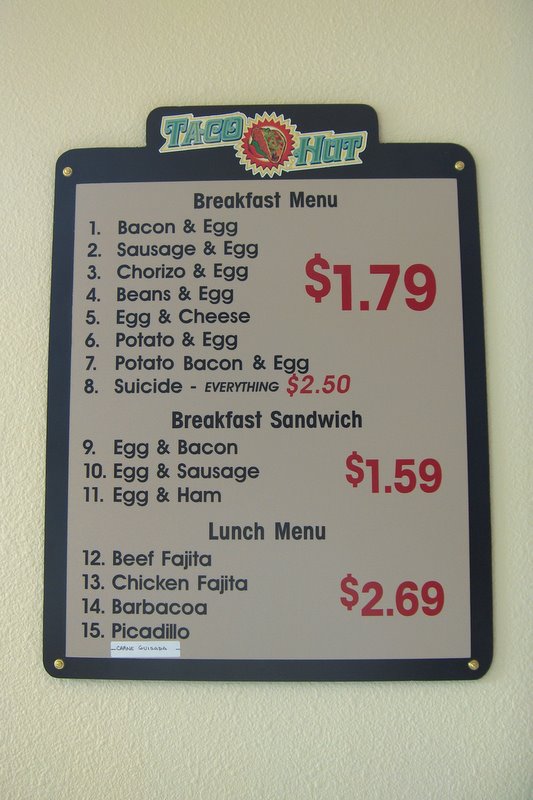The image captures an old, possibly outdated menu from a place called Taco Hut, which offers more than just Mexican cuisine. The menu is a single page, mounted on the wall, possibly pegged up with text. There is a "breakfast menu" section, where all items, including bacon and egg, sausage and egg, and chorizo and egg, are priced at $1.79 each. Additionally, there is a unique item labeled "Suicide," which costs $2.50 and contains all ingredients.

The menu also features a "breakfast sandwich" section, with each sandwich priced at $1.59. In the "lunch menu" section, options such as beef fajita and chicken fajita are listed, each costing $2.69. The price structure is simple and the prices are notably low, suggesting the menu might be from an earlier time.

At the bottom of the menu, there is an unreadable label mentioning a "carne" dish. The name starts with a "G" and it appears to have been added after the original menu was created.